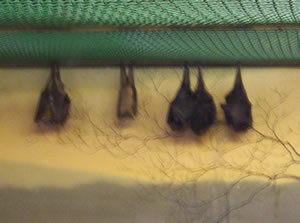The image depicts five small bats, all hanging upside down with their wings covering their bodies. They are arranged from left to right with varying spaces between them: a lone bat on the far left, followed by a single bat in the middle, and three bats clustered together towards the right. These bats appear black and are suspended from a material resembling a green fence or roofing, some parts appearing marbled and cracked. In the backdrop is a beige to dark yellow gradient, with the silhouette of a barren tree branch and a distant tree line or ridge.